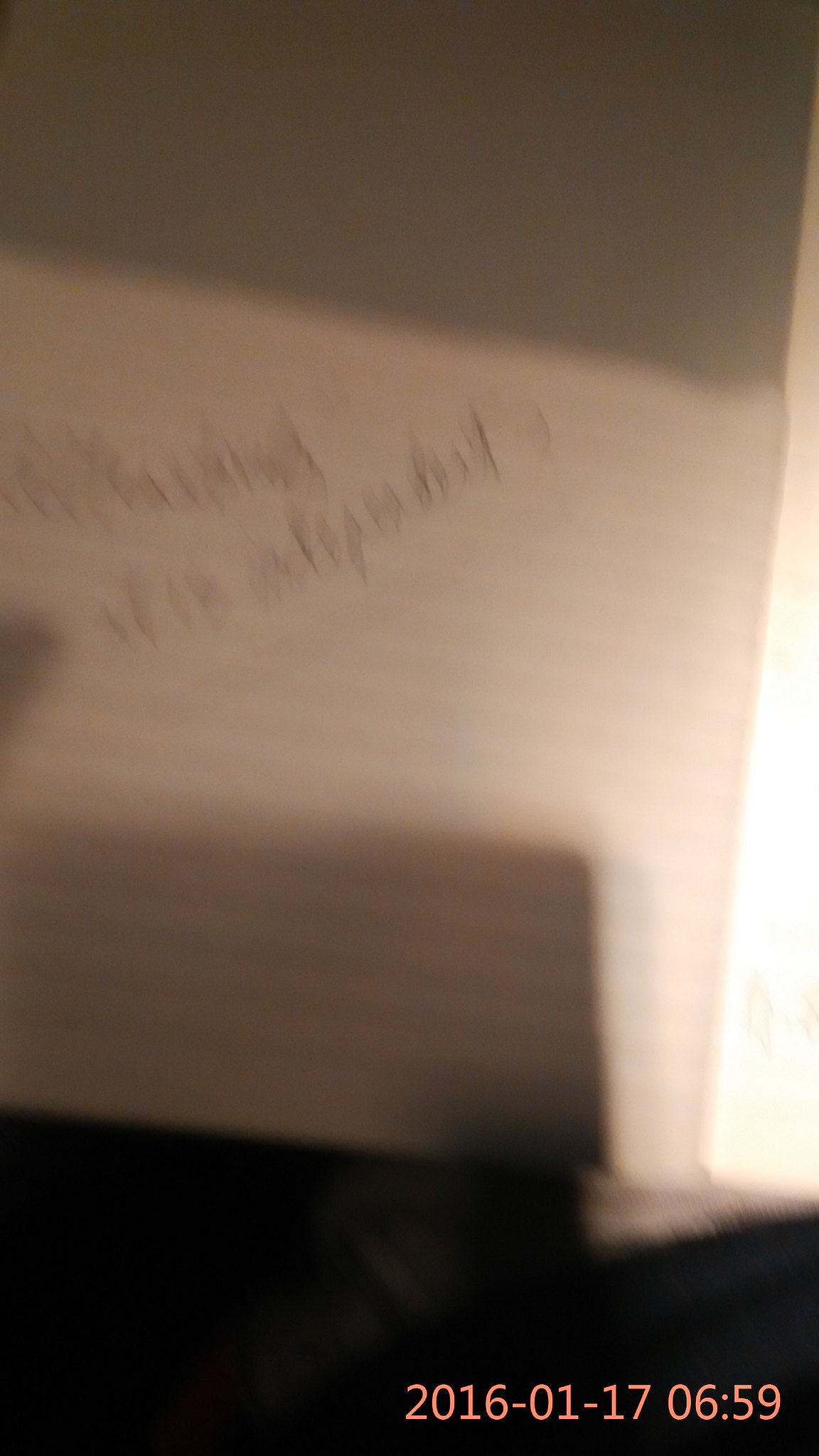This is an extremely blurry, low-resolution photograph of a piece of lined paper. The paper is pinkish due to the lighting, which shines from the right side and casts rectangular shadows across the top. The main focus is the handwritten text, written in cursive with a pencil, diagonally crossing multiple lines and underlined. The text appears to begin with "plus 18" followed by more cursive writing, though it's difficult to decipher due to the blur. In the middle of the image, a white, square-shaped object also displays two lines of text written in black. At the bottom right corner of the photo, in peach color, the date "2016-01-17" and time "06:59" are visible. The background includes a dark grayish fabric with potentially lighter material on top.